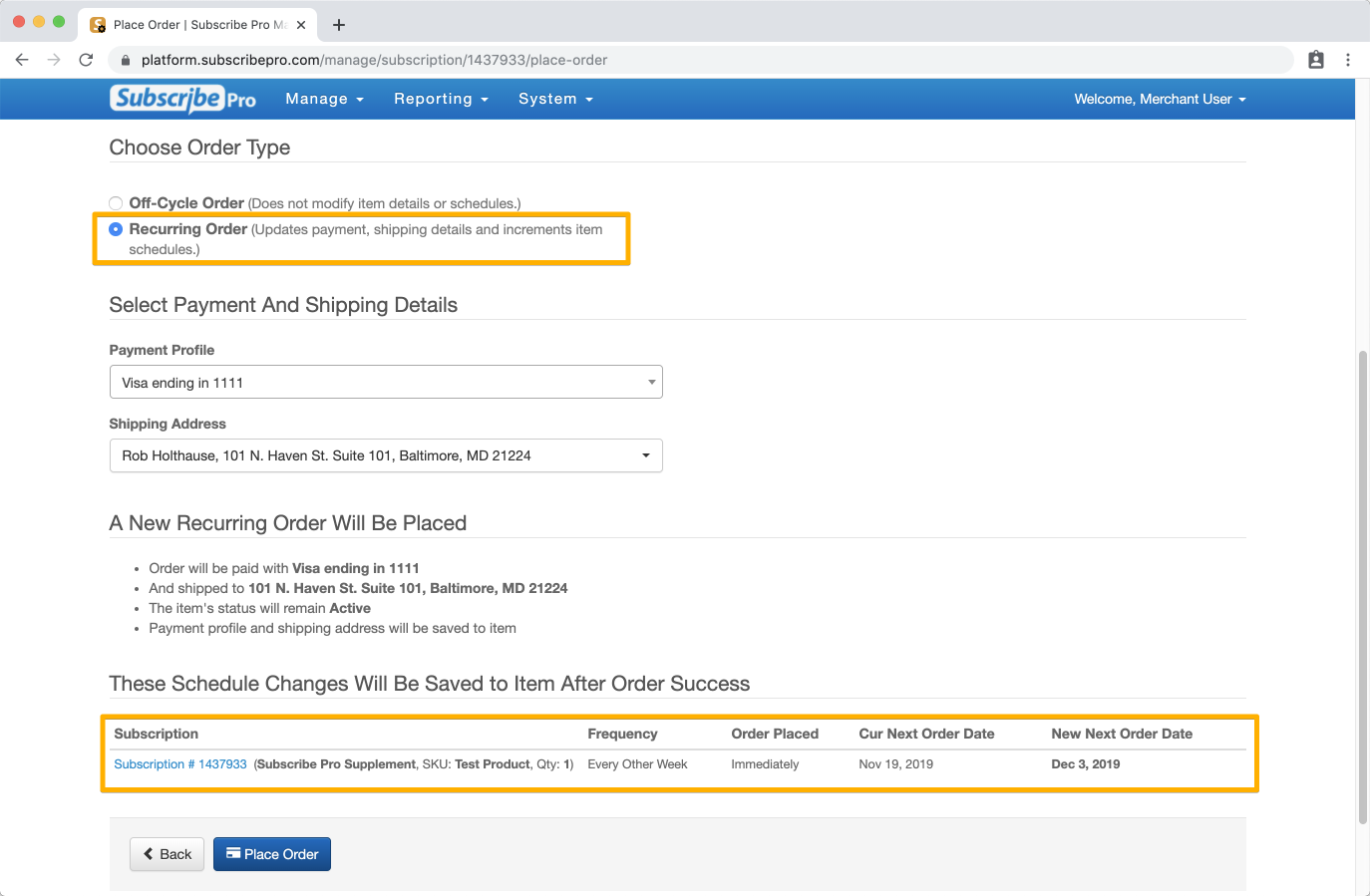A screenshot of a Google Chrome browser window, currently displaying an order page for Subscribe Pro. The interface features a blue navigation bar at the top with tabs labeled "Subscribe Pro," "Manage," "Reporting," and "Systems." Beneath this, the prompt to "Choose Order Type" is visible, with the "Recurring Order" option selected. Further down, sections for selecting payment and shipping details are shown, including options for a pre-saved credit card and a pre-saved shipping address. Below these sections, a message indicates that a new recurring order will be placed, accompanied by detailed information about the subscription.